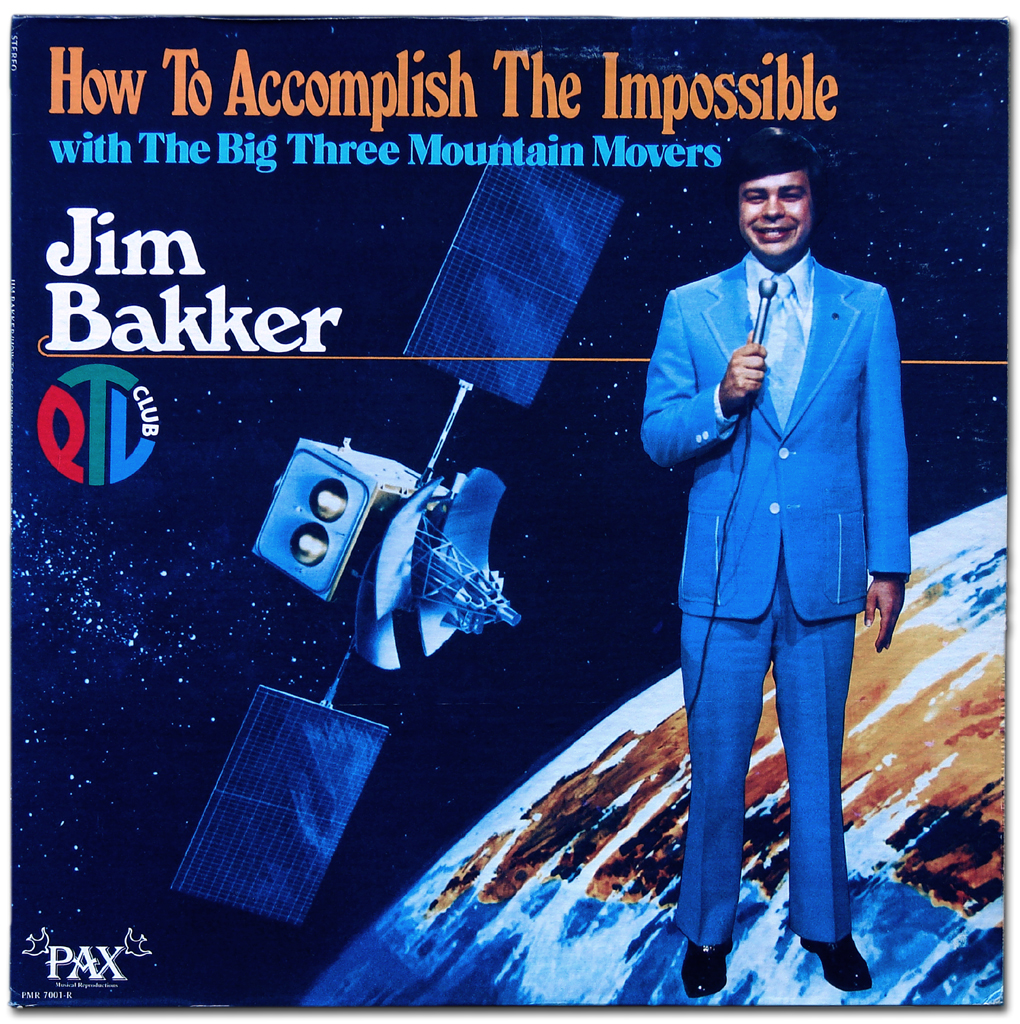In the image, a man, identified by text as Jim Baker, is standing upright in front of a space-themed backdrop. He is dressed in a medium blue, two-piece business suit, reminiscent of the 60s or 70s, complete with visible pockets on both sides of the coat and two buttons, of which the bottom button is unbuttoned. He also wears black business shoes and has dark brown hair, styled neatly. He's holding an old-fashioned wired microphone and is smiling slightly, showing a bit of his teeth, with his eyes appearing to squint.

The background reveals the dark expanse of space, scattered with stars, and prominently features a satellite angled to Jim’s left. At the bottom right, the Earth is visible with its atmospheric white blending into brown continents. The text on the image includes an orange headline reading "How to Accomplish the Impossible," with a subtitle in blue letters stating "With the Big Three Mountain Movers." Below this, "Jim Baker" is written in white, with a circular logo featuring red, green, and blue colors next to it, indicating "PTC Club." 

This meticulously arranged scene seems to be a digitally created graphic, highlighted by the mixture of space elements and text, suggesting a promotional theme.